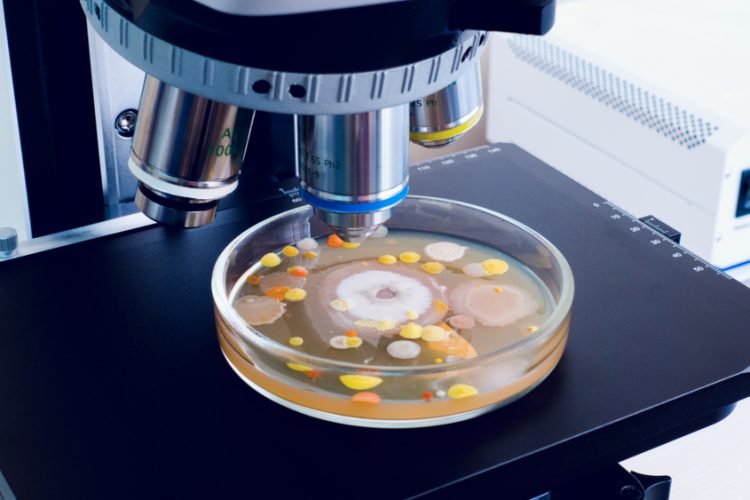This detailed color photograph, likely taken in a science lab or school classroom, captures a close-up view of a microscope's black base holding a clear Petri dish under one of its lenses. The microscope prominently displays three differently colored lenses—white, blue, and yellow. The Petri dish contains a clear gel-like liquid with various circular objects of multiple colors and sizes, including yellow, orange, red, and white, suggesting the presence of fungi, algae, or other microorganisms. The clear Petri dish reveals suspended round formations resembling globs and splatters. To the right of the microscope, a white radiator with lines of open spaces is partially visible, possibly indicating the image is set on a worktable.